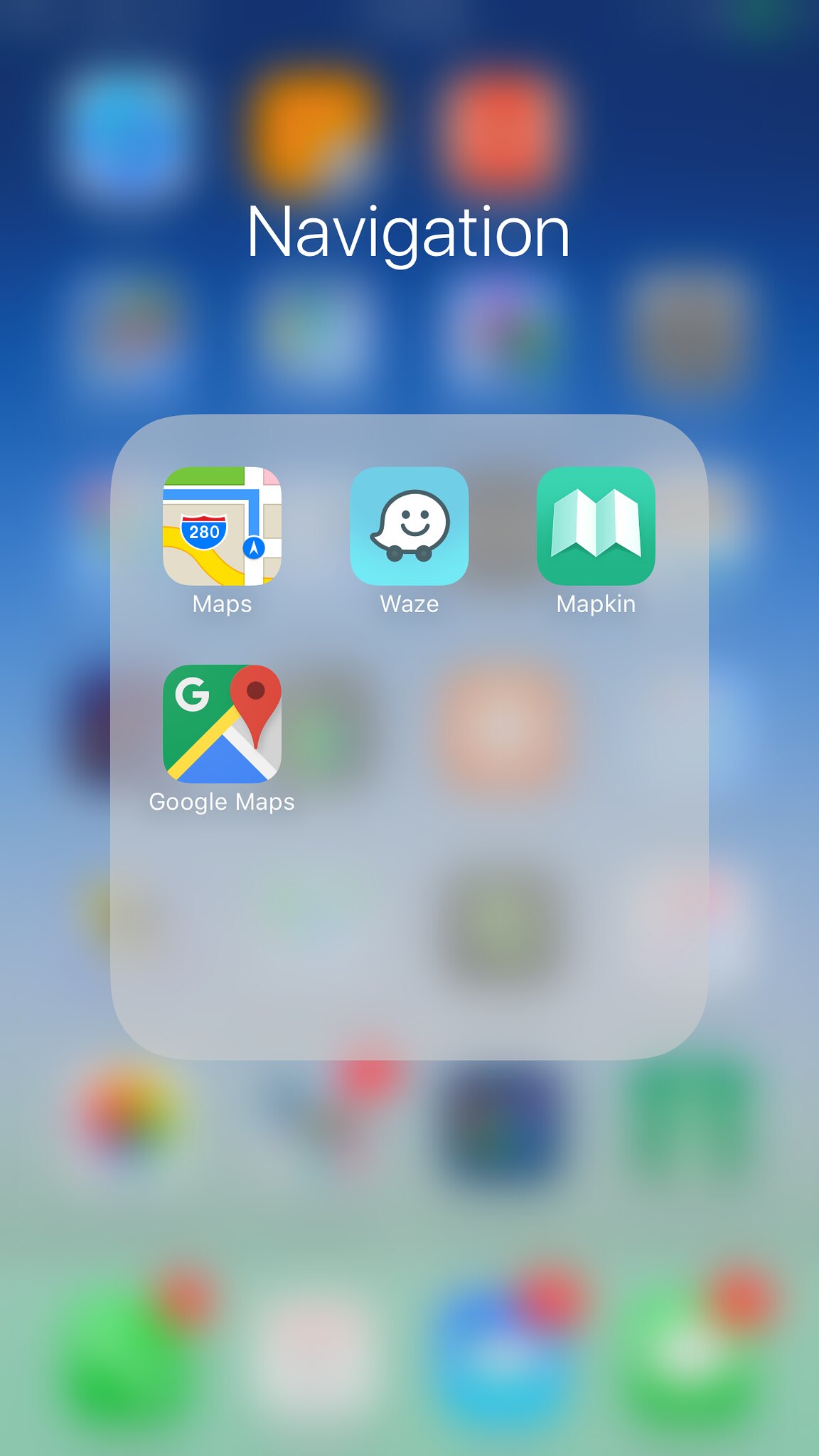The photo is a screenshot captured from an iPhone, showcasing the contents of a folder titled "Navigation." The title "Navigation" is displayed at the top in white lettering. Below the title, there is a semi-transparent, square box that houses four app icons arranged in a 2x2 grid, each representing a different navigation application.

1. **Apple Maps**: This icon features a multicolored representation of a map with a highway sign reading "280" and intersecting blue and yellow lines.
2. **Waze**: The Waze icon is a blue square with a white, smiling ghost figure that has two feet.
3. **Mapkin**: The Mapkin icon is a green square with a minimalist white line map.
4. **Google Maps**: This icon displays the iconic Google "G" on a colorful background, complete with a red location arrow and segments of yellow and blue.

The screenshot hints at the presence of other apps on the home screen, but they remain out of focus, making them indistinguishable.